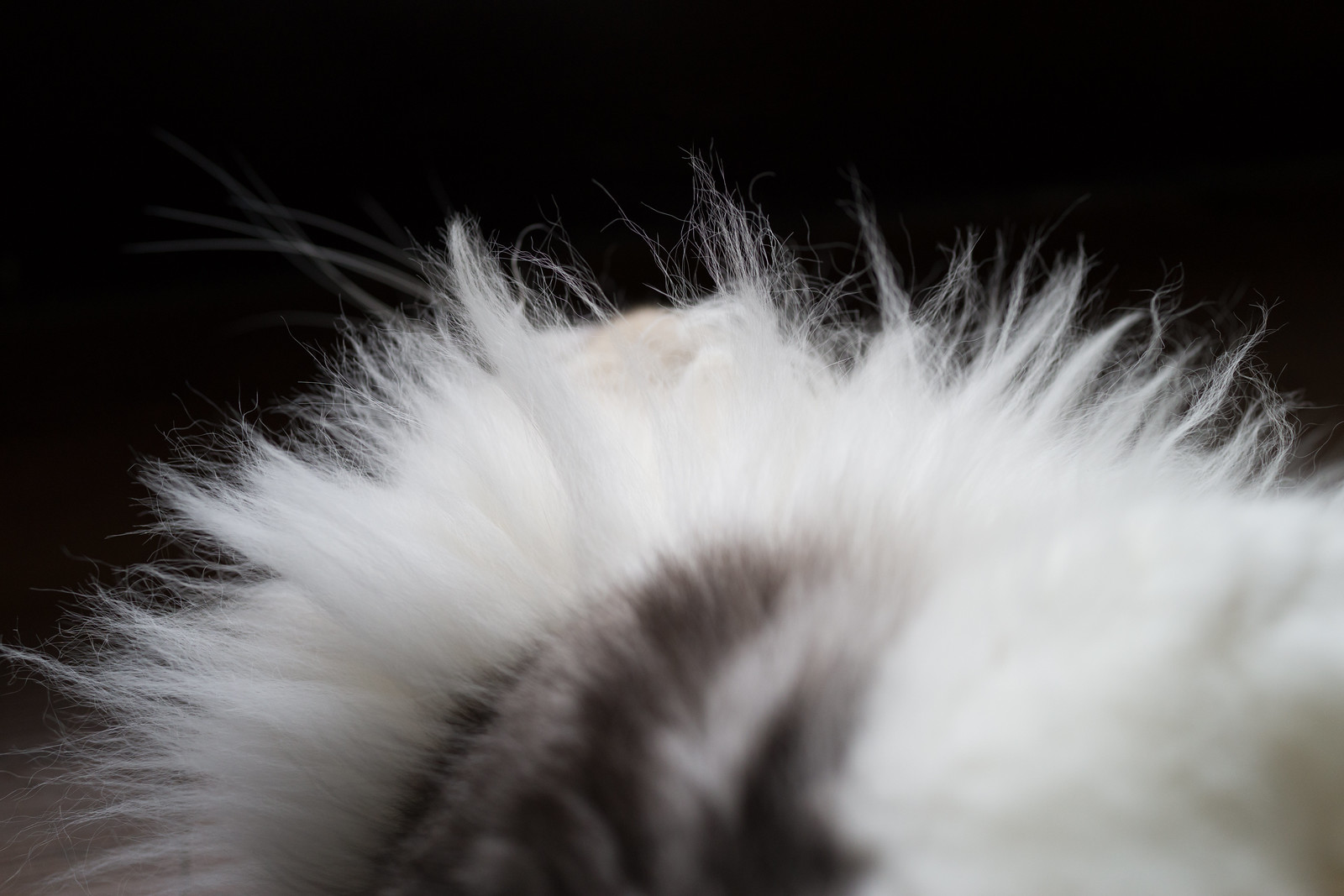The photograph, taken against a black background, captures a close-up view of fur, possibly that of an animal or an object made from fur. The fur is primarily white and stretches from the lower left corner of the image, rises up to the center, and then extends down to the lower right. A distinctive patch of black fur is noticeable towards the bottom center of the photo, creating a striking contrast with the surrounding white fur. The black and white colors are vivid and true-toned, with the background appearing dark and the fur at the back looking slightly blurred, emphasizing the fur in the foreground. The precise nature of the fur is unclear due to the image's hurried capture, but it might belong to an animal like a skunk or a cat, though this is not certain.